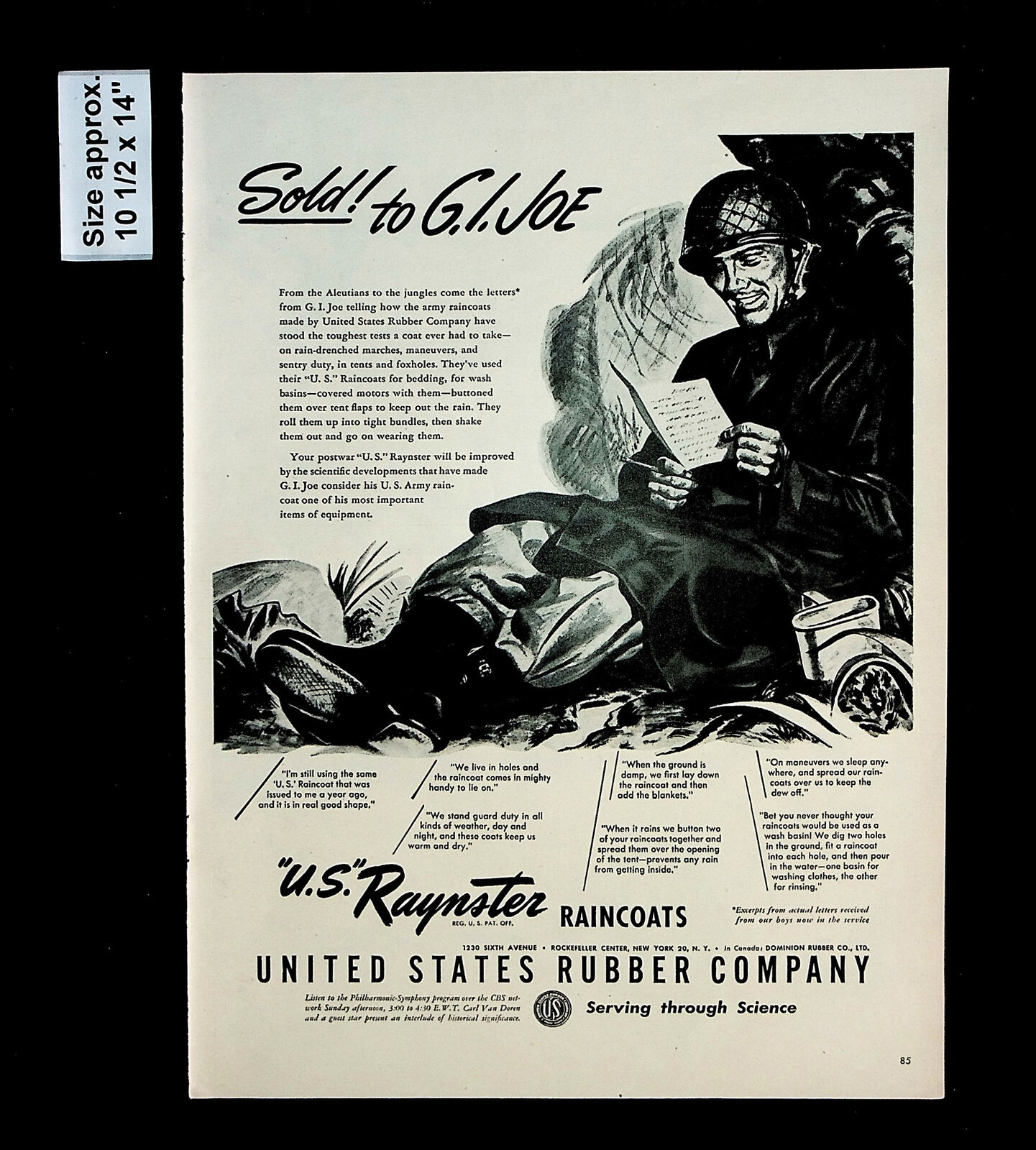This black-and-white vertically rectangular image appears to be an old advertisement or magazine page on slightly off-white paper. The most notable feature is a drawing of a World War II era soldier sitting and reading a booklet or letter, dressed in a helmet, dark coat, light pants, and boots. Situated in the upper left corner of the image, there is a small box with black text indicating the size of the page, approximately 10.5 by 14 inches, while the phrase "Sold to G.I. Joe" is prominently displayed nearby. Below the soldier’s drawing are several paragraphs of small, somewhat illegible text in quotes. At the bottom of the image, it reads “U.S. Rainster Raincoats, United States Rubber Company” followed by “Serving Through Science” in the lower right corner, where the page number "85" also appears, suggesting it might be from a magazine. The image is bordered by a thick black frame, particularly thicker on the left side.